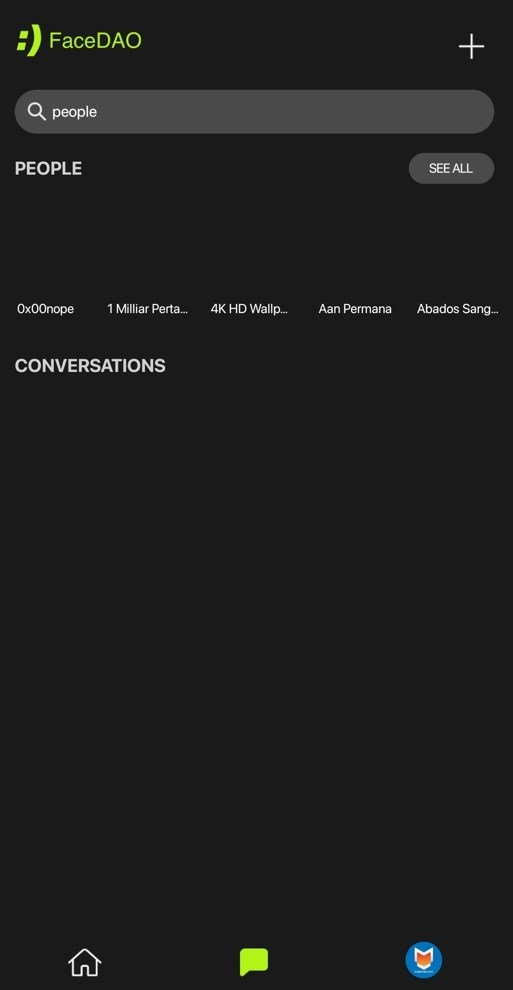The image appears to be a screenshot from a mobile phone interface featuring a predominantly black background with white text. In the upper left corner, there is a smiley-face emoticon made with a colon and parenthesis, followed by the word "FACEDAO" in lime green color. On the far right, a small white plus sign is visible. Beneath this, a large gray search bar is prominently featured, labeled "PEOPLE" in white capital letters, and underneath this is the word "PEOPLE" again in white. To the right of the search bar, there is a gray button with the text "SEE ALL" in white.

Further down, there is a section that appears to be divided and labeled with various terms including "XOXOO," "1 Miller Porta 4K HD wallpaper," "AANPERMA," "ABADOS," and "SANG." Below this section, the word "CONVERSATIONS" is displayed in white capital letters. The majority of the remaining area below this label is black, empty space. Finally, at the bottom of the image, there are three graphical icons: a white house symbol on the left, a lime green conversation bubble in the center, and a blue circle on the right with a red object in the middle, resembling a notification or alert.